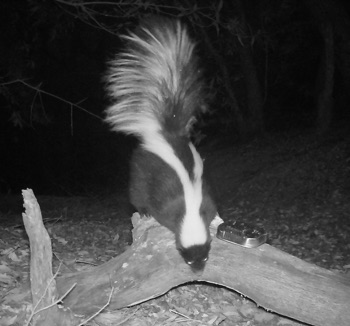In this detailed nighttime photograph, a skunk stands on a large, rough-hewn tree limb or piece of driftwood set against a pitch-black backdrop. The flash or additional nighttime lighting used to capture the scene accentuates the skunk's striking black and white markings. The skunk, illuminated in the darkness, reveals a stunning contrast of colors: an all-white head, a white stripe that divides into a V shape mid-back, and a bushy tail that is predominantly black with grayish-white tips. The tail is raised high, suggesting the skunk is either alert or potentially in a defensive posture. The skunk's eyes gleam in the light, adding a touch of eerie brilliance. There appears to be a metallic object, possibly a container, near the tree limb, though its specific details are indistinguishable. The backdrop hints at an outdoor setting, possibly a sandy area or a forest clearing, completing the striking nocturnal scene.